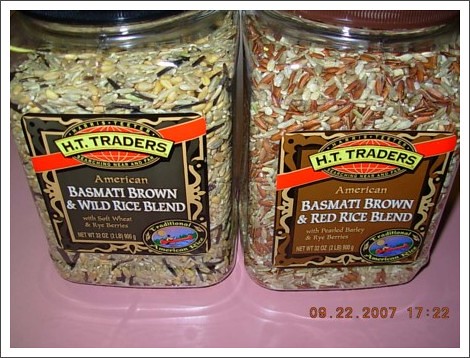This photograph features two clear, upright plastic canisters with large, circular lids, each containing a different type of rice blend. 

- The canister on the left holds a mix of black, white, and off-white/yellowish rice varieties. It is labeled "HT Traders American Basmati Rice and Wild Rice Blend."
- The canister on the right contains a blend of white and reddish-brown rice, labeled "HT Traders American Basmati Brown and Red Rice Blend."

Both containers rest on a mauve or lavender-purple surface. In the bottom right-hand corner, the image is timestamped with "09.22.2007 17:22," indicating the date and time the photograph was taken.